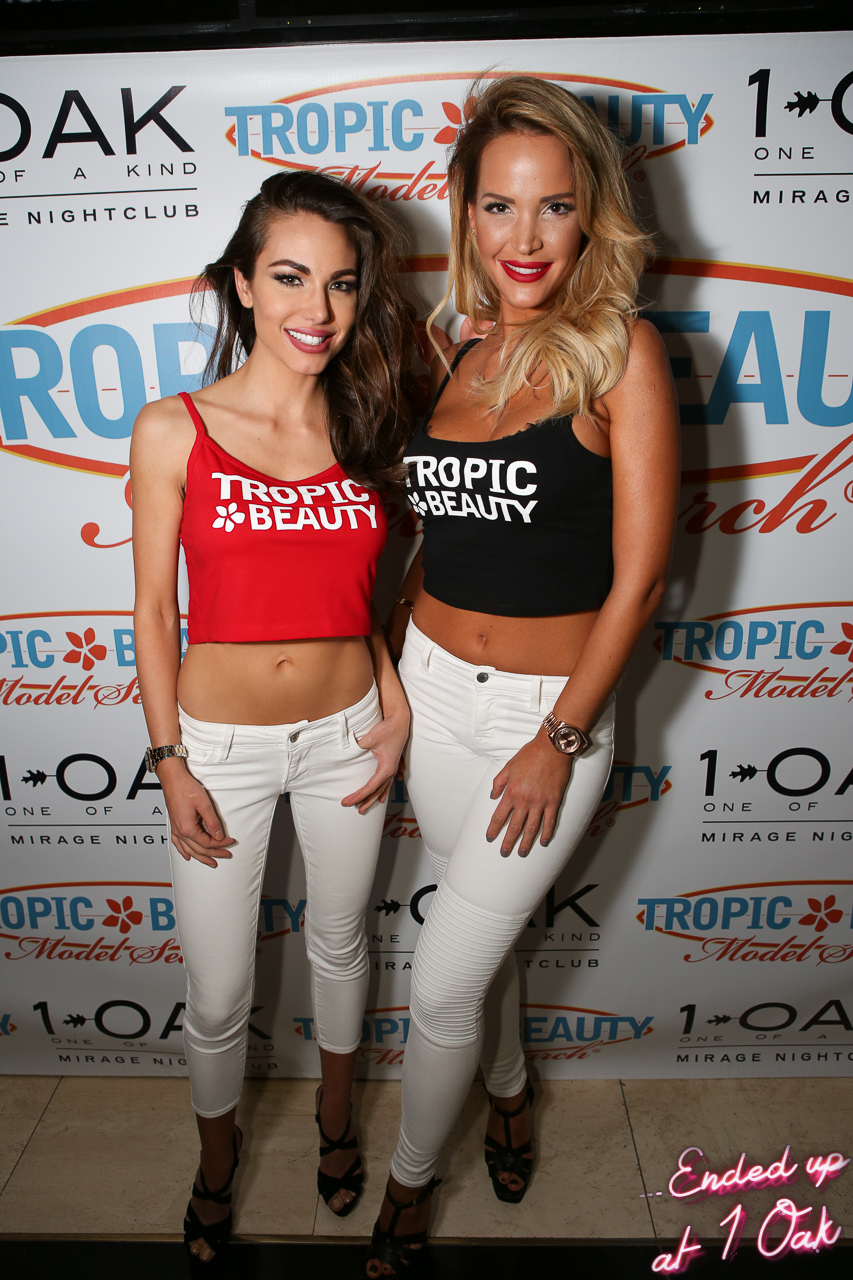In the photograph, two women, both wearing cropped tank tops and white skinny jeans, are posing. The woman on the left has dark brown hair, a bright red tank top with "Tropic Beauty" and a flower in white font, low-rise cropped white skinny jeans, and black heels. The blonde woman on the right, who is taller, wears a black tank top with "Tropic Beauty" in white font, ankle-length white skinny jeans, and black heels. They are standing on a tile floor in front of a white event advertisement sign featuring logos and text for "One Oak," "Mirage Nightclub," and "Tropic Beauty." At the bottom of the sign, in a neon-like cursive font, it says "ended up at One Oak."